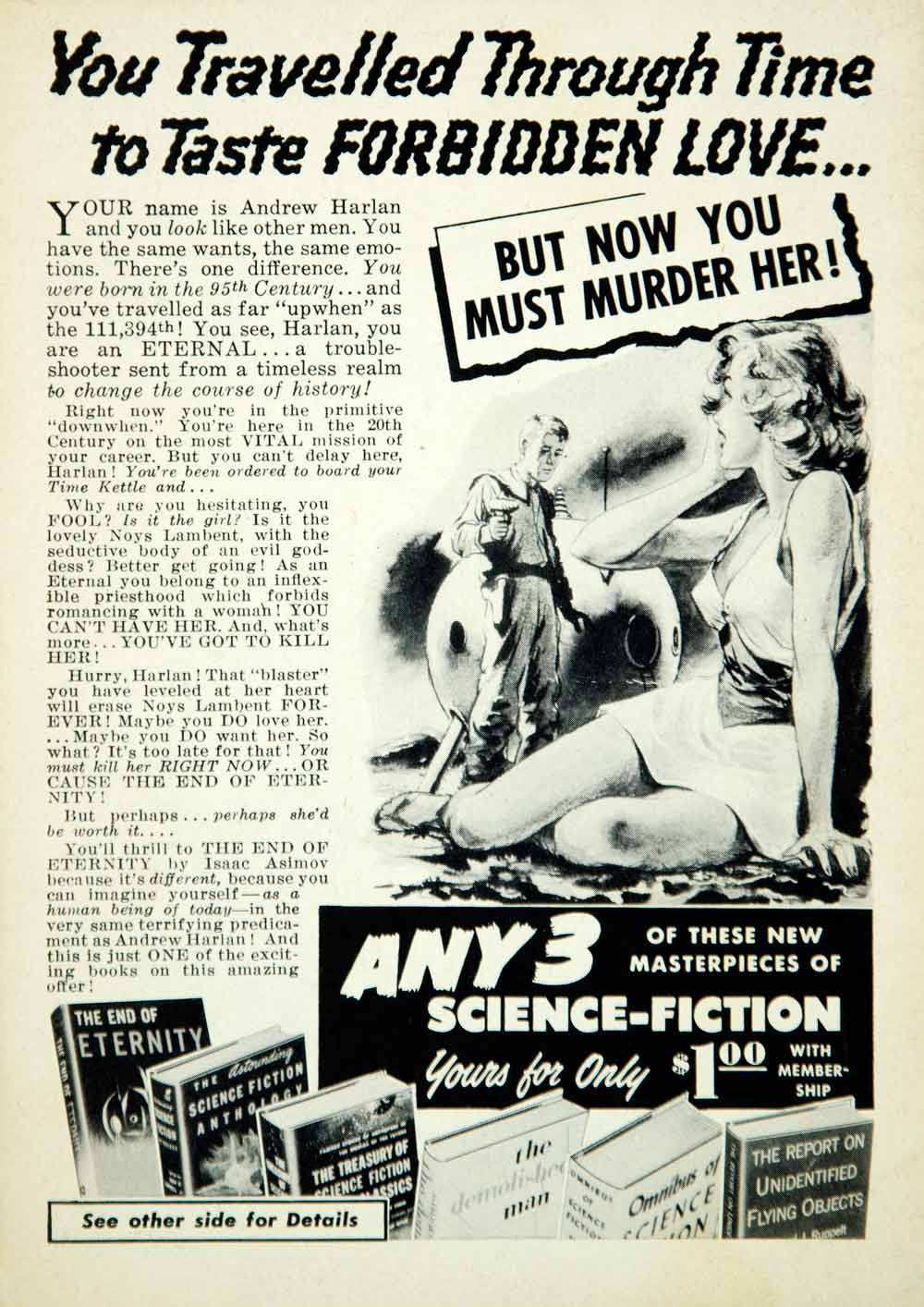This black and white vertical image appears to be a vintage magazine advertisement, resembling an old newspaper ad in style. The center features a dramatic scene: a woman in a provocative, short skirt and low-cut blouse sits on the ground, her blonde hair flowing. She rests her right hand thoughtfully under her chin while her left hand is placed beside her. Standing over her is a man clad in what appears to be a space suit, holding a gun. Behind him, a round object with landing gears and portholes, likely a spacecraft, is visible. 

Above this scene, bold black letters convey a suspenseful narrative: "You traveled through time to taste forbidden love... but now you must murder her." Below the image, a promotional offer reads, "Any three of these new masterpieces of science fiction, yours for only $1 with membership," accompanied by book titles like "The End of Eternity," "Science Fiction Anthology," and "The Treasury of Science Fiction Forensics.” The overall layout and artistic style give this ad a distinctly retro, science fiction allure.